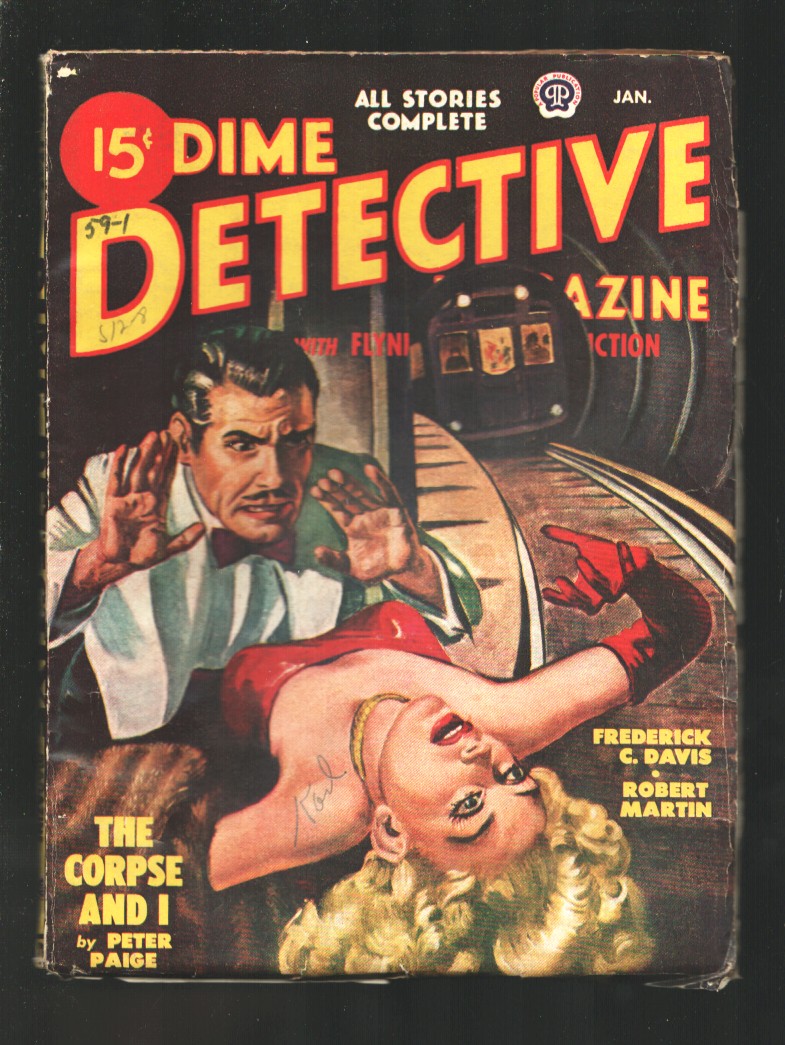The image depicts the cover of a vintage comic book titled "15 Cent Dime Detective Magazine." Dominated by a dramatic film noir style, the cover features a black background and vivid red and yellow lettering at the top proclaiming "15 Cents" and "Dime Detective Magazine," with the subtitle "All Stories Complete." Central to the illustration is a tense scene set in a subway station. A woman with blonde hair, a red dress, red gloves, a gold necklace, and a fur coat is perilously draped over train tracks. Her arms are outstretched as she appears to fall backward, while an oncoming train, filled with visible passengers, hurtles towards her. Above her stands a man dressed in a white tuxedo with a red bow tie and slicked-back black hair, sporting a 1920s-style mustache. His hands are raised near his face, seemingly in an attempt to reach for the woman. At the bottom of the cover, the feature story is titled "The Corpse and I" by Peter Page, Frederick C. Davis, and Robert Martin. The magazine also includes a date notation and Carl's signature, suggesting it was issued in January, with the code "S 12 8 59-1" incorporated into the design.